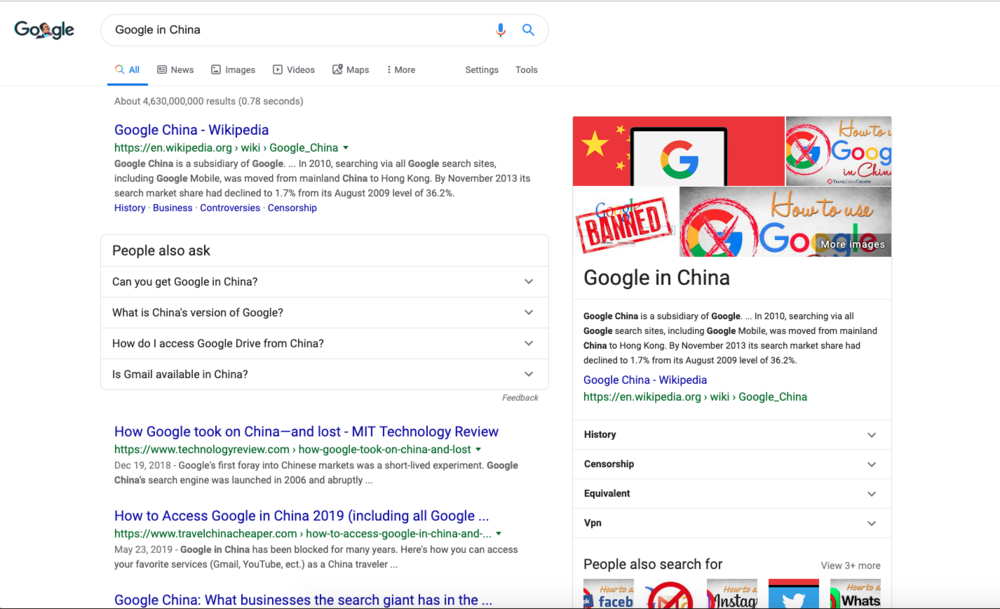A detailed article headline appears on a computer screen, addressing the impact of Google's operation in China. The search queries displayed on the screen cover various topics related to Google in China, including its history, market share statistics, and methods to access Google services within China. The screen shows a white background with a black line at the bottom, and there are multiple search result snippets from sources like Wikipedia and MIT Technology Review. The image captures a moment frozen in time where one is exploring Google's tumultuous journey in China and seeking detailed information on how the tech giant managed to navigate the restrictive digital landscape of the country.